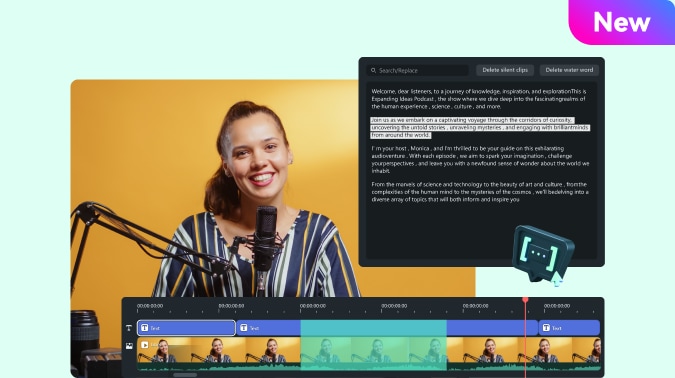The screenshot displays a sleek interface of a modern website, featuring a welcoming image of a young woman against a vibrant yellow background. She is seated confidently in front of a microphone, offering a warm smile to the camera. Her dark hair is neatly pulled back, and she dons a stylish vertically-striped shirt in shades of blue, white, and yellow. 

To the right of her image, a prominent black box contains partially legible text that begins with "Welcome to a journey of knowledge..." and continues with additional, indecipherable text, hinting at an educational or informative nature.

The bottom section of the screenshot showcases a horizontal gallery populated with thumbnail images of the woman, each set against the same yellow background. These thumbnails likely represent different segments of a video, allowing users to click and navigate to specific parts of the audiovisual content.

In the upper right corner of the screenshot, a visually distinct purple and blue box marked "NEW" captures the viewer's attention, suggesting recent updates or new content available on the website.

Framing the entire screenshot is a sea-green border, adding a refreshing and cohesive touch to the overall design.